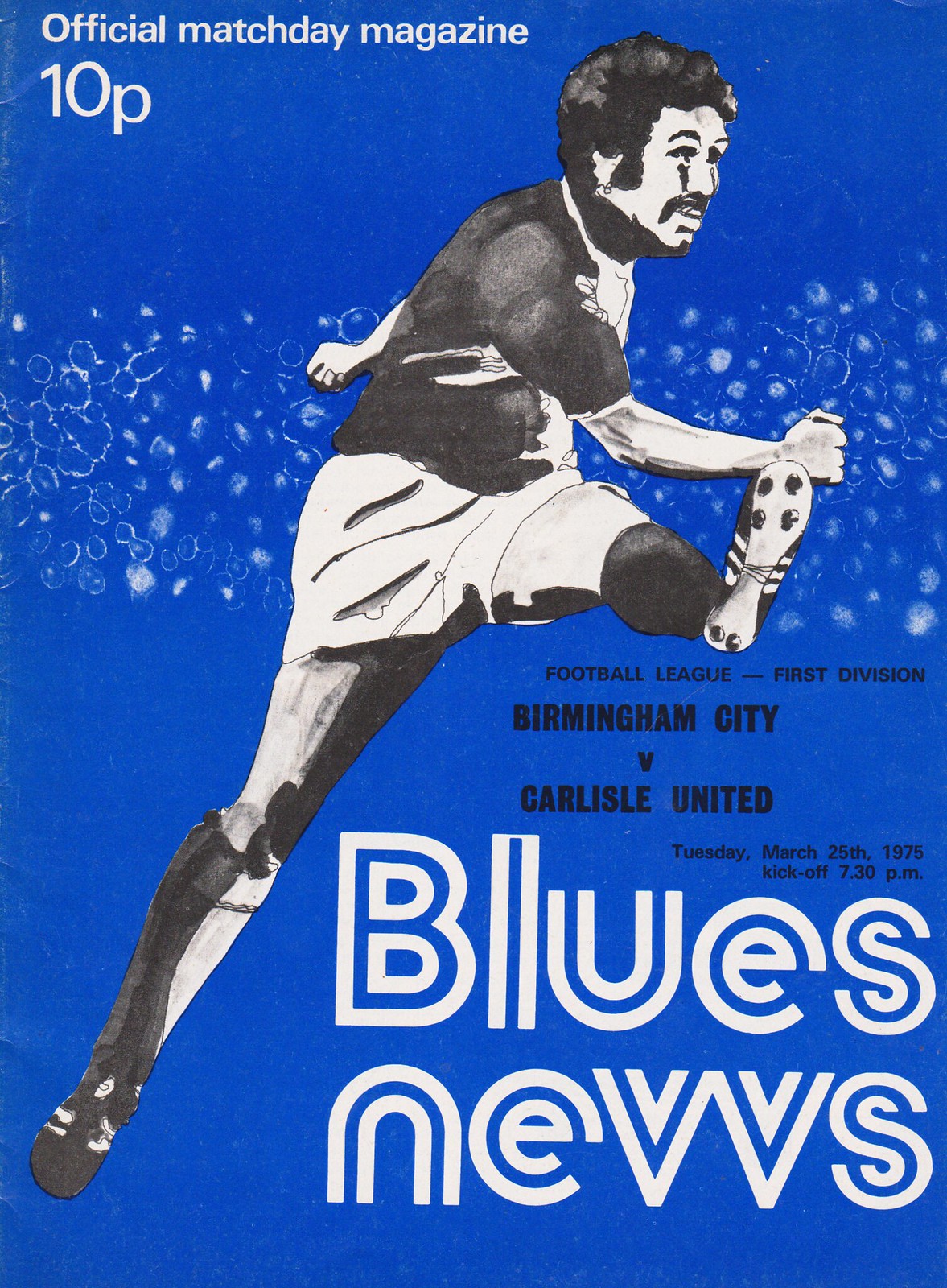This image showcases a scanned copy of an official Match Day magazine set against a striking blue background. Prominently, the top left corner features the text "Official Match Day Magazine 10P" in white font. Dominating the center is a large, hand-drawn, black-and-white graphic of a soccer player mid-kick. The player, depicted with black hair and possibly a mustache, is in motion with his left leg high in the air and his right arm crossed over his body. He dons a dark jersey, light shorts, cleats, and knee socks, embodying the intense energy of the sport. At the bottom right, large white text with a double border spells out "Blues News." Below this, in black font, are the event details: "Football League, First Division, Birmingham City vs. Carlisle United, Tuesday, March 25, 1975, Kickoff at 7.30 P.M." The entire backdrop is interspersed with smoky, white spots that create a cosmic, asteroid belt-like effect, adding depth and intrigue to the overall design.